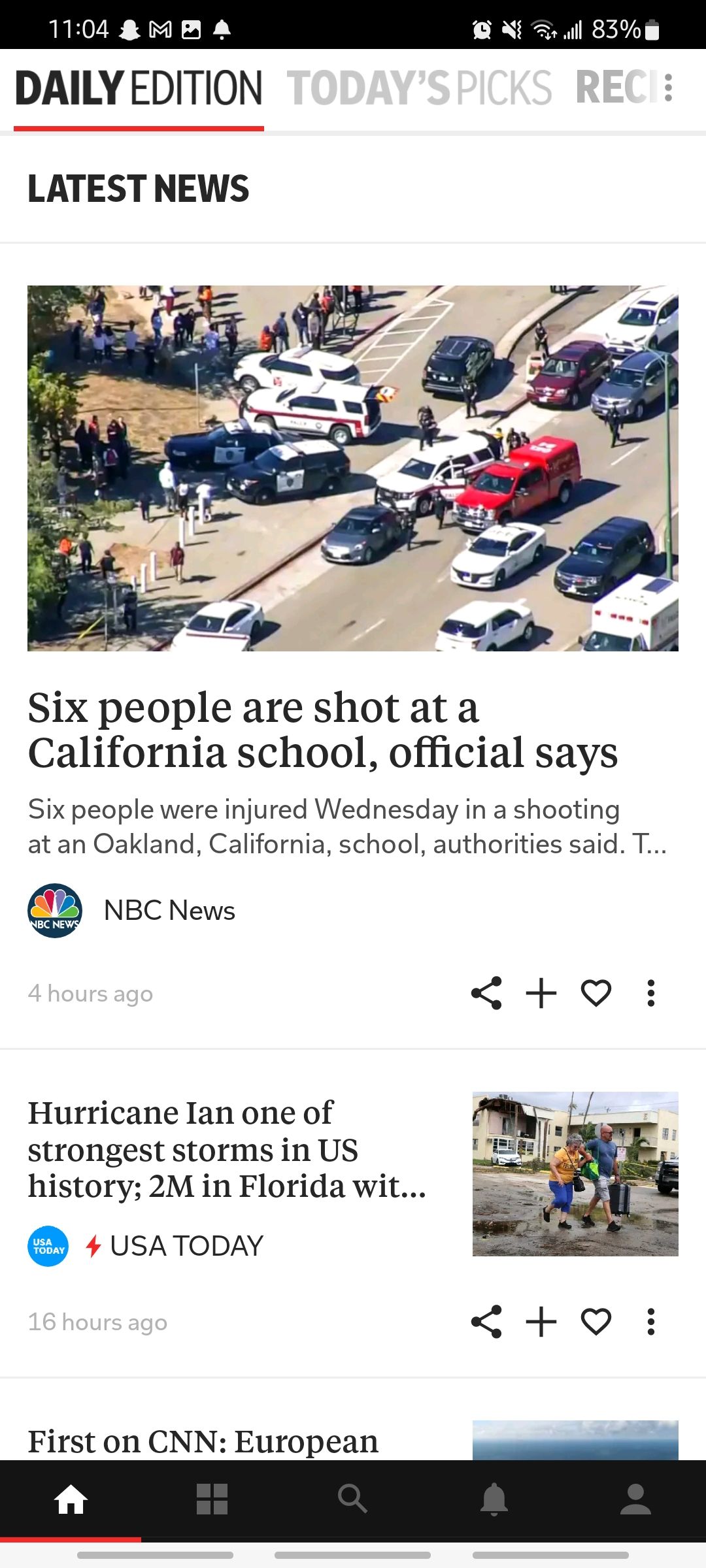The screenshot depicts a smartphone interface with a black header at the top. In white font, the time is displayed as 11:04, and on the right side, there is an 83% charged battery icon, a Wi-Fi icon, a wireless connection icon, a mute icon, and an alarm clock icon. Below the header, the website headline reads "Daily Edition" with a gray subheadline "Today's Pick." The remaining letters "REC" are partially visible on the right side.

Below these texts, the section "Latest News" is prominently featured with a large photo spanning the width of the screen. The overhead image shows numerous mostly white vehicles, which appear to be police cars, and pedestrians on the side of a street.

The main headline reads, "Six people are shot at a California school, official says." The subsequent headline underneath reads, "Hurricane Ian, one of the strongest storms in US history, affects 2 million in Florida," though the complete text is partially cut off. To the right of this text is a smaller photo of two white men carrying equipment with what looks like an apartment building in the background. The street in the image appears flooded.